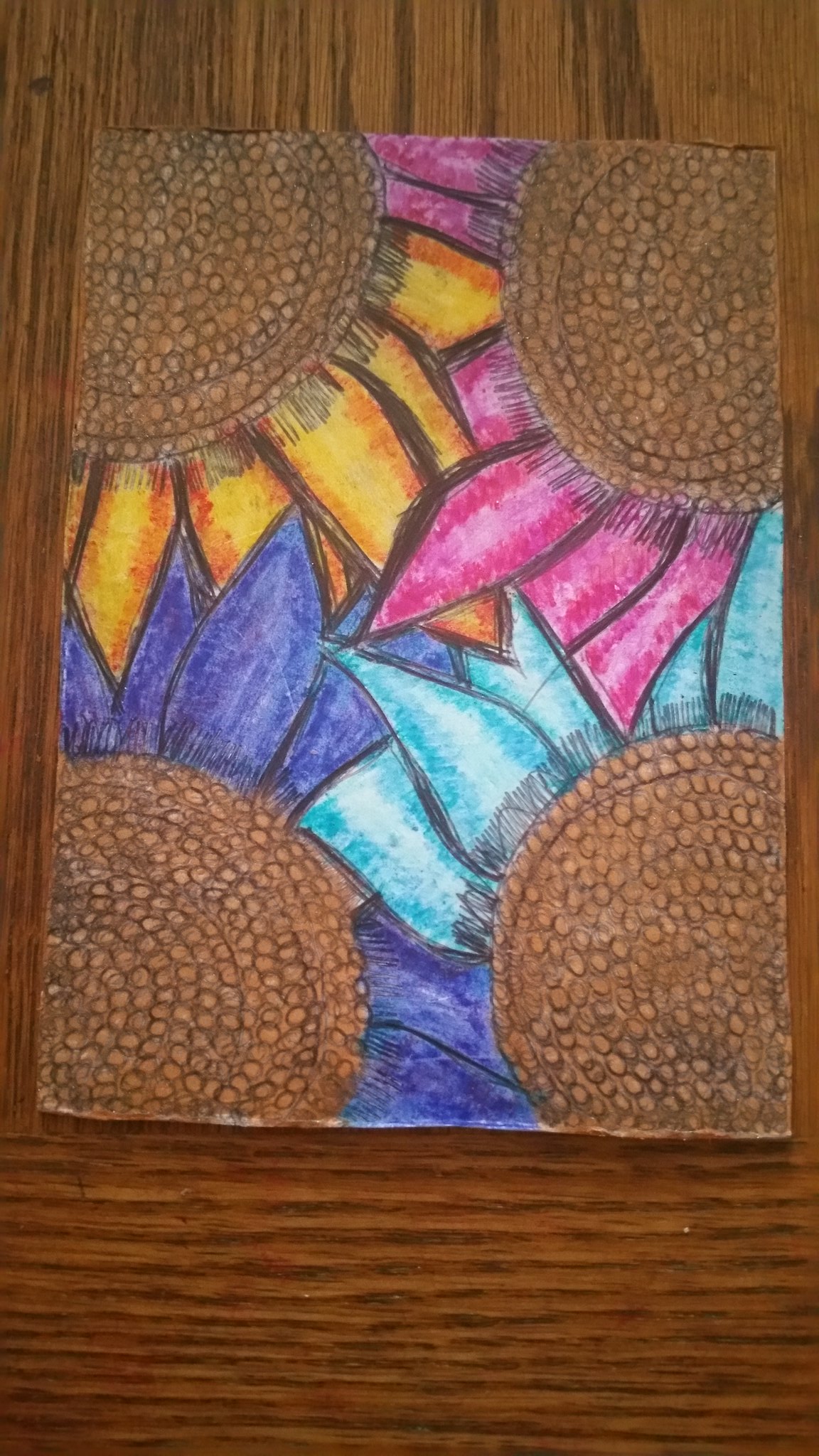This photograph captures a piece of art lying on a dark brown, golden-hued wooden table. The art features four large, overlapping flower petals rendered in shades of magenta, orange, dark blue, and light blue. Each petal is detailed with lighter bands of shading in corresponding hues, such as lighter pink, orange, and teal. The centers of the flowers are adorned with tan, nubby-like objects, resembling large sunflower centers, each intricately detailed with fine black lines reminiscent of black eyelashes. The black detailing continues around the edges of the petals, providing a crisp, defined look. In each corner of the artwork, these tan centers are circled with ricotta-colored accents, juxtaposing the vivid colors of the petals. This detailed and vibrant piece sits elegantly on a richly textured wooden surface, completing the composition.